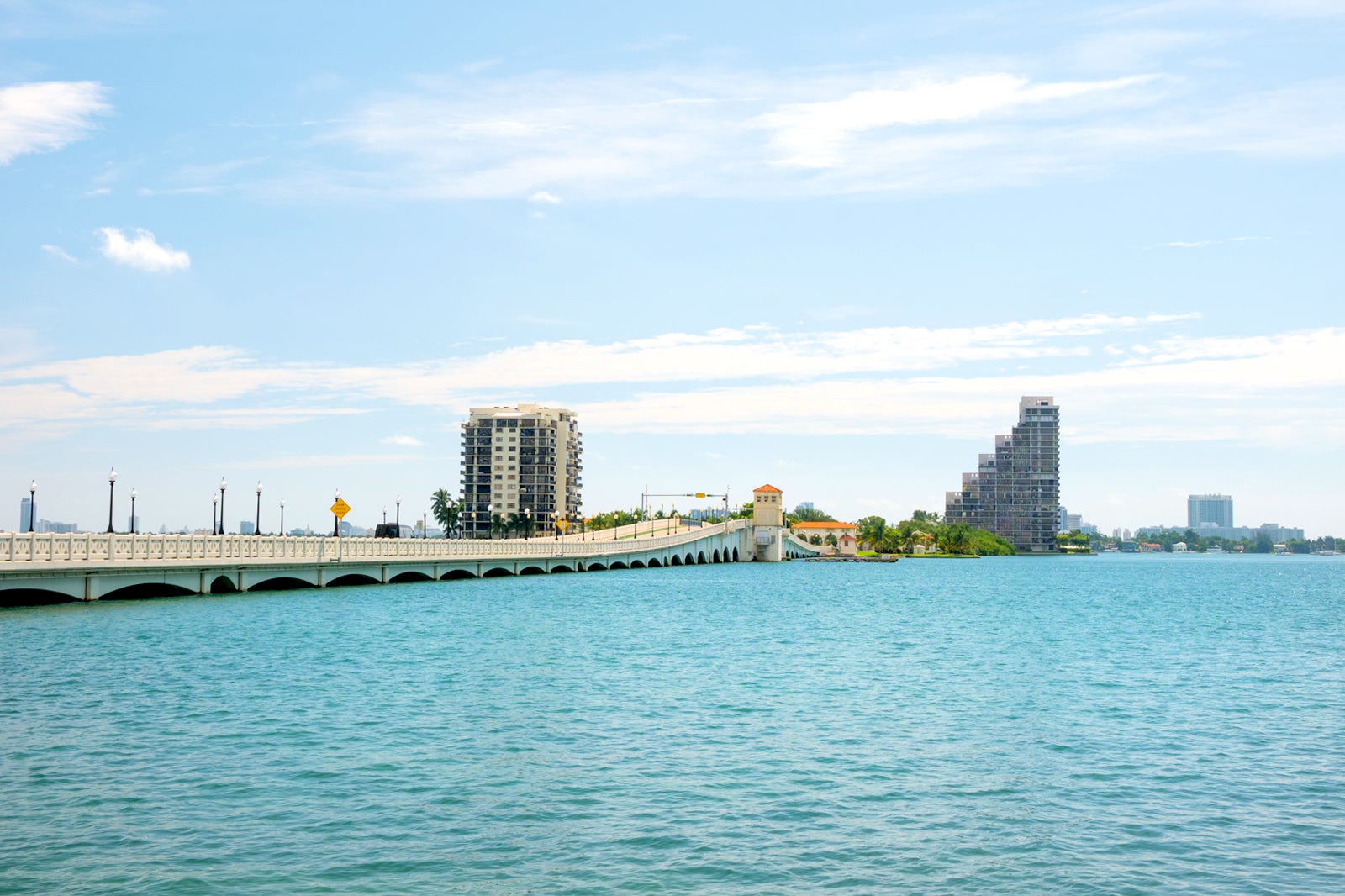This professional color photograph features the Venetian Bridge crossing a large, tranquil body of water that could be a lake or river. The crystal-clear blue water seamlessly blends with the vibrant blue sky, dotted with fluffy white clouds. The bridge, constructed of concrete and adorned with white railings, stretches from the center left into a bustling cityscape. It is lined with black streetlamp posts and features low arches. A terracotta-roofed tower stands prominently at one end, near the shore. In the background, a variety of large buildings and skyscrapers rise against the skyline. To the left, there is a very large hotel with 15 to 20 stories. Nearby, a peculiar skyscraper looms, with sections that increase in height like a staircase. Further left, more buildings, including an apartment complex with black, gray, and sandy-colored rectangular sections, are visible. The shoreline is dotted with trees and homes, adding a touch of greenery to the scene. A single black car is seen crossing the bridge, which also features yellow triangular street signs and a height warning sign at its entrance.